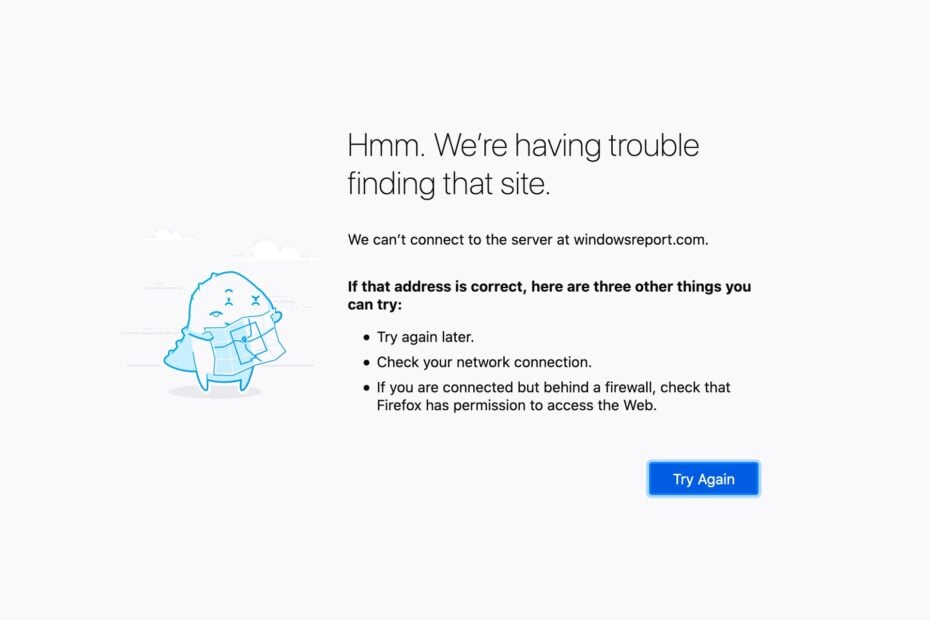This image is a screenshot from a website displaying an error message typically seen when encountering connectivity issues on Google. The screen has a clean, white background with large, central black text that reads, "Hmm. We’re having trouble finding that site." Below this, the message continues to specify, "You can't connect to the server at windowssupport.com. If that address is correct, here are three other things you can try."

The suggested troubleshooting steps are presented as bullet points:
1. Try again later.
2. Check your network connection.
3. If you are connected but behind a firewall, ensure that Firefox has permission to access the web.

On the right side of the error message is a prominent blue button with white text that says "Try Again." On the left, there is a small, whimsical cartoon character outlined in blue. This character has an upside-down head with closed eyes, small arms, tiny legs, and appears to be wearing a scarf. Its exasperated expression humorously embodies the frustration of not being able to connect to a website, a sentiment many can relate to. The context of this screenshot highlights the user’s personal experience of having to switch from a slow mobile broadband connection to a slightly more reliable phone connection, in hopes of avoiding this very issue.